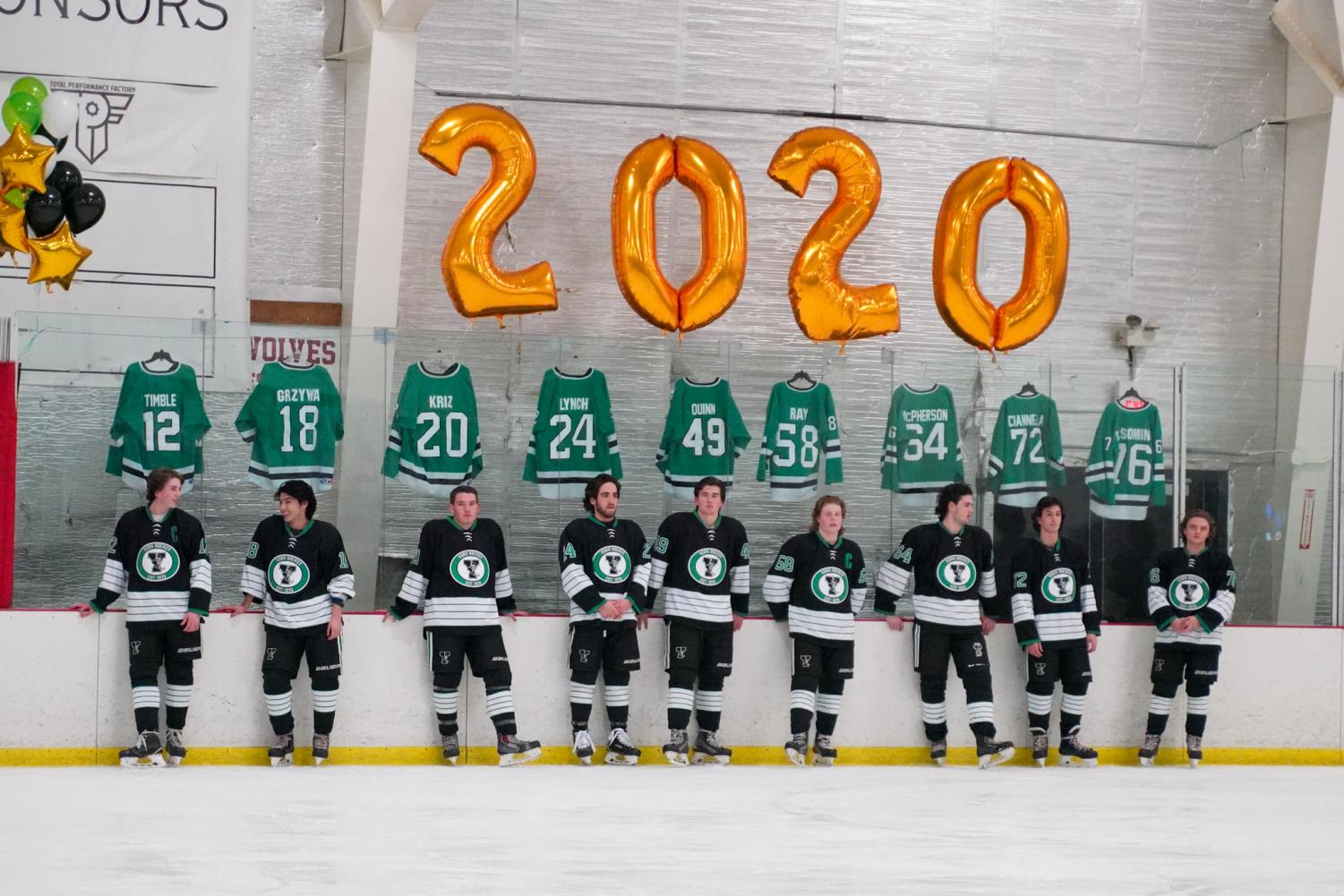This landscape-oriented photograph captures a hockey team posing on an ice rink. The bottom 20% of the image showcases the white ice, meeting a rink wall bordered by a yellow strip. Above the yellow strip, the wall is predominantly white with a small red trim at the top. Leaning against this wall in a row are approximately ten Caucasian male hockey players, all dressed in matching black jerseys, shorts, and black and white socks, with their uniforms accented by white and green elements. Positioned above them, displayed prominently, are their green jerseys featuring their names and numbers, such as Timmel (#12) and Ray (#58). Towering above the jerseys are gold balloons forming the year "2020," alongside additional gold, green, and black balloons in the upper left-hand corner. The background of the scene is a silvery-gray wall, completing the backdrop for this team portrait, which marks the year they took this commemorative photo. The jerseys also feature a distinctive "Y" logo, adding a unique touch to the team's uniform.